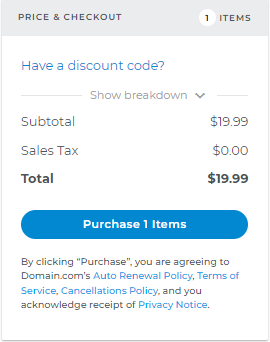In the image, the background is white, creating a clean and simple look. At the top of the image, there is a light blue rectangular box with the text "Price and Checkout" prominently displayed. Within this box, a white circle contains the number "1," indicating the presence of one item in the cart.

Below the "Price and Checkout" header, the word "Items" is written, followed by a blue-colored text inviting users to "Have a discount code?" There is a clickable line labeled "Show breakdown," accompanied by a small downward arrow icon.

A detailed breakdown follows:
- **Subtotal**: $19.99
- **Sales Tax**: $0.00
- **Total**: $19.99

At the bottom, there is a blue button with white text stating "Purchase 1 items." Beneath this button, there is a disclaimer in smaller font. It reads: "By clicking Purchase, you are agreeing to Domain.com's auto-renewal policy, terms of service, cancellations policy, and you acknowledge receipt of the privacy notice." Some of this text is highlighted in blue, indicating clickable links.

Overall, the image conveys the final steps of an online checkout process, emphasizing the purchase total, the option to enter a discount code, and the agreement to the website's terms and policies.